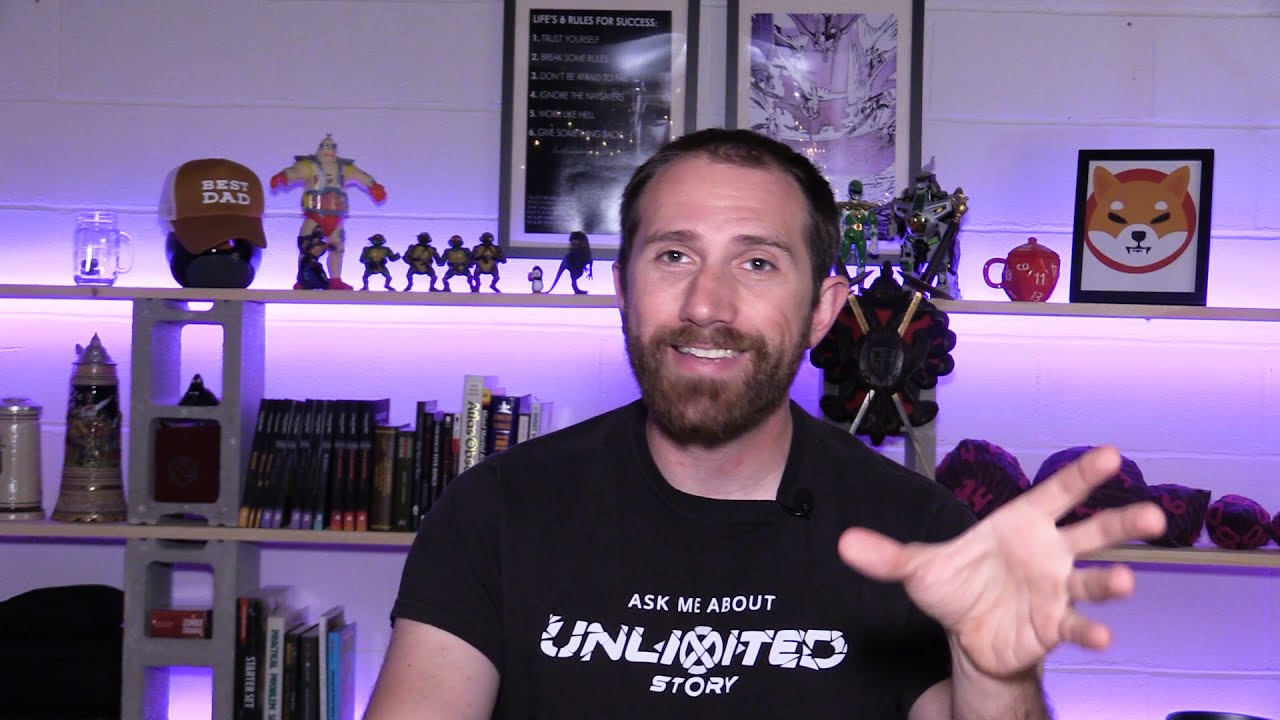The image portrays a man, potentially in his early to mid-30s, with a short dark beard and short hair. He is facing forward with his eyes looking slightly to the left of the viewer, and he has a slight smile revealing his top teeth. The man is wearing a black short-sleeved t-shirt with white text that reads "ask me about Unlexited story." His left hand is raised and extended outward, as if gesturing while speaking. Behind him is a cinder block shelf adorned with various items: a hat that reads "best dad," action figures including the Teenage Mutant Ninja Turtles, a dinosaur, a penguin, a green Power Ranger, and a sword. There is also a red coffee cup shaped like a 20-sided die, several books, a cartoon image of a dog, and some stuffed plushies resembling dice. The background appears to be indoor, featuring a cement wall with pictures and lighting beneath the shelves, adding hues of brown, off-white, black, orange, red, yellow, light purple, dark purple, and blue to the scene.